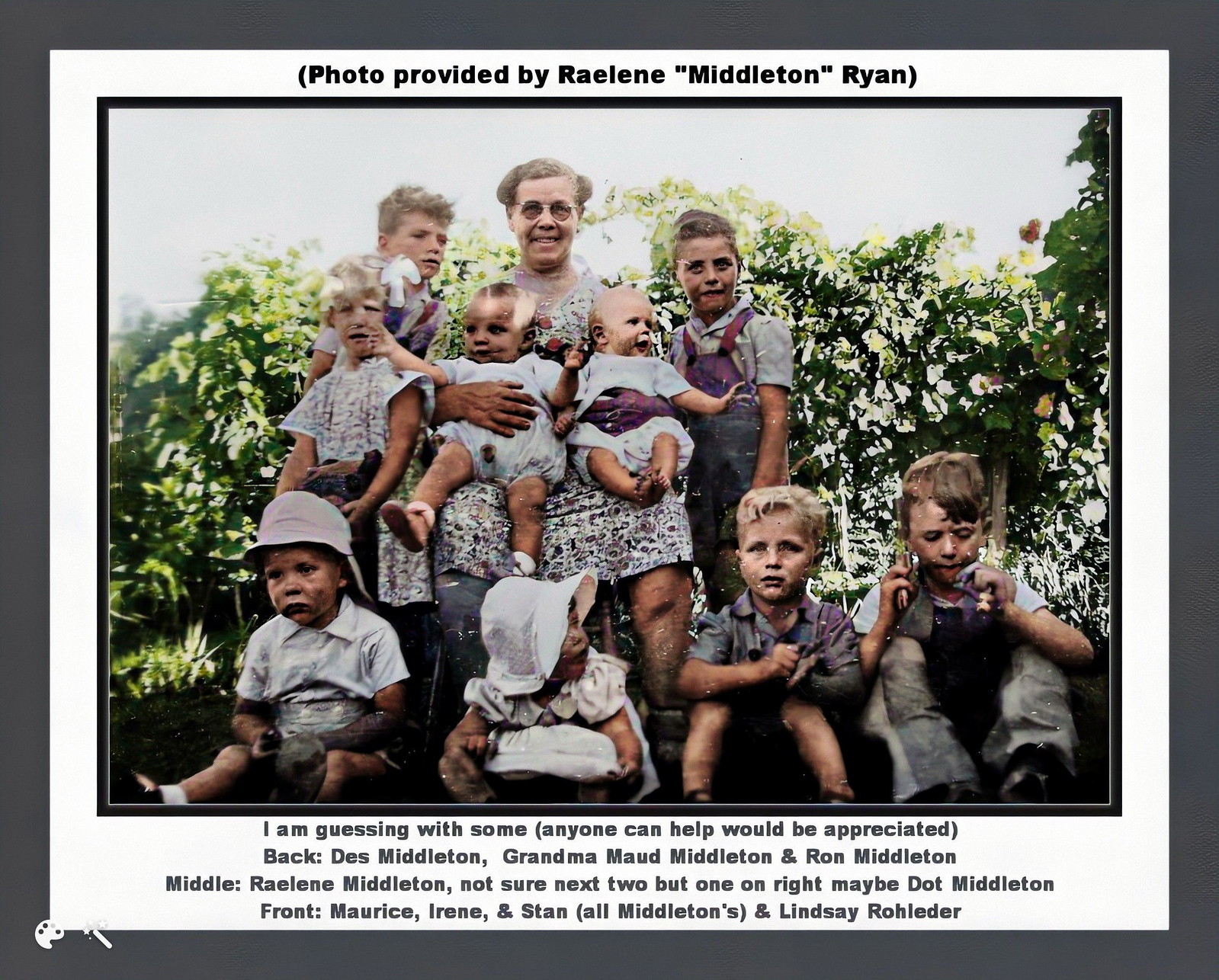In this charming black-and-white family photo, Grandma Maude Middleton stands in the center, lovingly holding two infant babies, one in each arm. Surrounding her are nine children, presumably her grandchildren, dressed in similar hues of purple, white, and gray. Immediately to her left and right are two older boys donning overalls, likely Des and Ron Middleton. To her left stands a girl adorned with ribbons in her hair, possibly Raylene Middleton. Down in front, four more children sit on the ground. From left to right, these include Maurice, Irene, and Stan Middleton, along with another child who could be Lindsey Roldor. The children range in age from as young as four months to approximately ten years old. They are posed in front of a verdant landscape of trees, suggesting a garden or farm setting, under a bright yet overcast sky. Above the image, the caption reads, "Photo provided by Raylene Middleton Ryan." Below, there's also text seeking identification assistance, which reads: "I am guessing with some, anyone can help would be appreciated. Back: Des Middleton, Grandma Maude Middleton, and Ron Middleton. Middle: Raylene Middleton. Not sure next to (her), but one on right may be Dot Middleton. Front: Maurice, Irene, and Stan (all Middletons), and Lindsey Roldor."